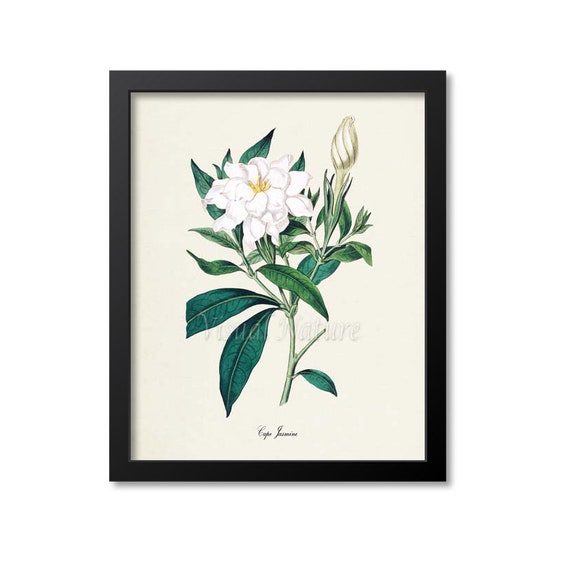This image showcases a black-framed print hung on a white wall, creating a stark contrast against the background. The artwork inside the frame features a cream backdrop, prominently displaying a large white flower with yellow in the middle. Surrounding the flower are vibrant green leaves and a green stem, adding a touch of nature's freshness. To the right of the fully bloomed flower, there is a bud that has yet to open, hinting at the promise of future blossoms. The painting is subtly overlaid with the text "visual nature" running across the middle, blending seamlessly with the soft tones of the artwork. At the bottom of the print, there's a partially legible signature, where the second word reads "jasmine," though the first word remains unclear. The delicate interplay of white petals and cream hints beneath them enriches the visual depth of the flower.